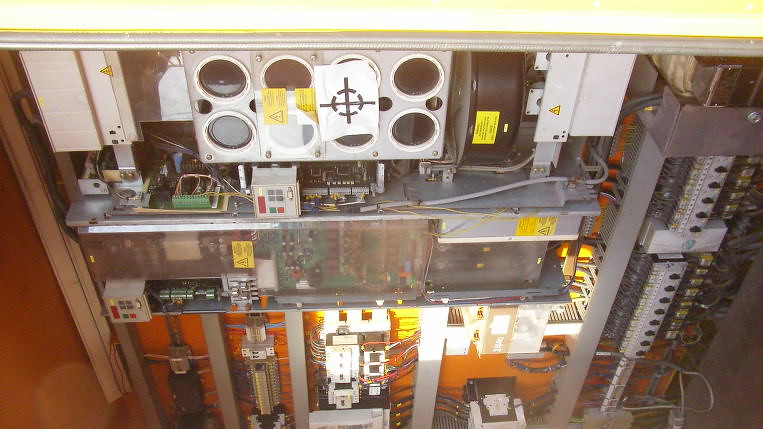The photograph depicts the intricate inner workings of an aged electrical system, illuminated by a yellowish filter that suggests the image has some age. Dominating the right side, multiple vertically-aligned, white, box-like breakers are neatly set within a metallic frame. Each breaker features a small black button and is connected to numerous organized wires extending outwards. Above these breakers, horizontally-arranged dual circular gauges are visible, adorned with paper displaying target symbols. Beneath this area lie extensive and colorful circuitry and PCB boards, intricately wired and painted in diverse hues such as green, blue, brown, and various metallic shades. The bottom section showcases a complex arrangement of vertically-installed electrical transformers and circuits. The entire setup is interspersed with vibrant yellow warning labels, and additional white and red stickers, all against a striking red backdrop, creating a vivid and detailed representation of this electrical unit, possibly within a server room environment.